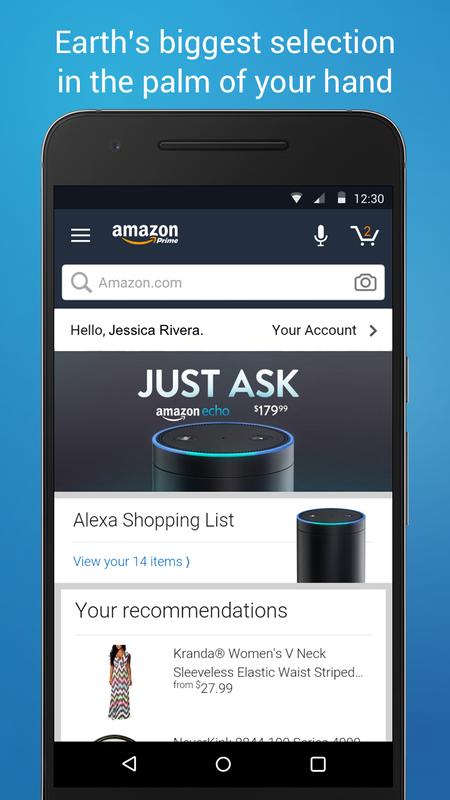This vertically-oriented image features a smartphone set against a serene blue background, which transitions subtly from a lighter hue at the top to a slightly darker shade at the bottom. The background showcases a smooth texture with minimal contrast. 

At the top center of the image, the phrase "Earth's biggest selection in the palm of your hand" is displayed in white text. Below this text, a black-rimmed iPhone is prominently featured, displaying an Amazon app page.

On the Amazon app interface, the icon for additional options, represented by three white bars, is located on the left-hand side. On the right, there are icons for a microphone and a shopping cart, the latter indicating that it contains two items. At the top of the screen, indicators show the time (12:30), the battery life, and several triangular signal strength icons.

Located at the top of the display is the Amazon search bar, which includes a small camera icon. Just below the search bar, the text "Hello, Jessica Rivera" is visible, along with options to access her account details. There is also a promotional banner offering the Amazon Echo at $179.99, and a section for the Alexa shopping list, indicating that there are 14 items that can be viewed.

Finally, beneath the shopping list, the app shows personalized recommendations and a series of navigation icons along a black bar at the bottom of the screen.